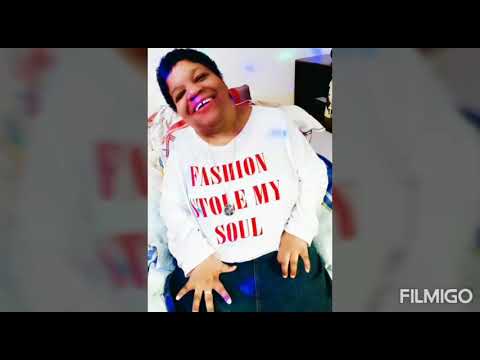In this vibrant image, the main focus is an African-American woman with short black hair, sitting down and radiating joy with a broad smile, showcasing a small gap between her front teeth. She is clad in a white shirt emblazoned with red text reading "Fashion Stole My Soul." Her lower attire appears to be either blue jeans or a blue skirt, complemented by a ring on her finger. She strikes an expressive pose with one hand resting delicately on her lap, and the other forming a dynamic gesture with her fingers splayed. Behind her, a white wall forms the backdrop, with a black table or shelves visible in the upper right-hand corner. The image has a distinct look, possibly due to damage or a light effect scattering blue orbs across it. The photo also features black framing at the top and bottom and a logo in the lower right corner that says "film ago." The color palette includes white, red, black, blue, and hints of brown, pink, and purple, enhancing the overall composition.